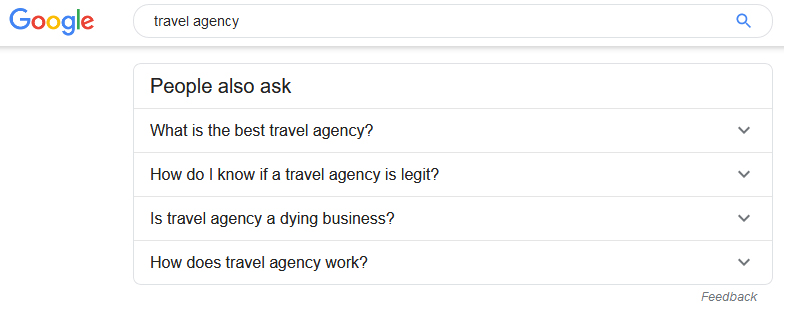The image portrays a web browser screenshot showing the top portion of a Google search results page. The area is approximately two and a half to three times as wide as it is tall. In the upper left corner, the iconic Google logo is prominently displayed. To the right of the logo, the Google search bar extends, occupying around 80% of the width across the top. The search query "travel agency" is typed in black, lowercase text within the search bar. At the far right end of the search bar, there's a blue magnifying glass icon.

The background throughout the entire image is a clean, unbroken white, giving no distinct viewable edges to the screenshot. Directly beneath the search bar, there's a light gray horizontal bar. Below this bar, several rectangular query boxes are aligned sequentially.

Each box starts in alignment with the gray bar above and is separated by a light gray line. The boxes are stacked vertically and contain popular related queries:

1. "People also ask"
2. "What is the best travel agency?" with a down arrow on the far right
3. "How do I know if a travel agency is legit?" also accompanied by a down arrow on the far right
4. "Is travel agency a dying business?" again with a down arrow on the far right
5. "How does travel agency work?" with a down arrow on the far right

At the very bottom right corner of the last query box, there is italicized, gray text reading "Feedback."